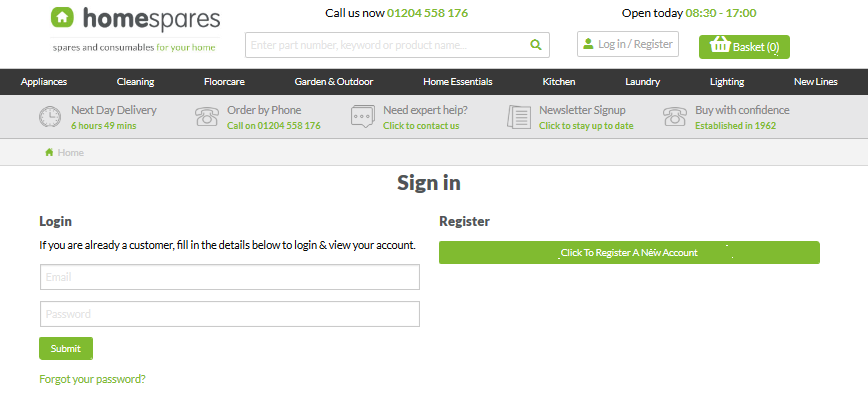In the image, the top section features a header titled "home spares" in all lowercase black letters. To the left of the text is a small green box with a house icon inside. Below this header, a tagline reads, "spans of commutes for your home." To the right of "home spares," there is a "callers now" prompt displaying the phone number 0-1-2-0-4-5-5-8-1-7-6. Further to the right, another section indicates the business hours with "open today, 8:30 to 17:00" (5:00 p.m.).

Beneath the "callers now" prompt, there's a search bar adorned with a magnifying glass icon. Adjacent to the search bar are options for "login/register" with an associated icon, and a shopping basket icon displaying a "0" in parentheses. Underneath this is a navigation bar with menu options: "appliances," "cleaning," "floor care," "garden and outdoor," "home essentials," "kitchen," "laundry," "lighting," and "new lines." This bar is highlighted with a black background.

Next, a gray text bar lists services: "next day delivery," "order by phone," "need export help," "newsletter sign-up," and "buy with confidence." Below, in green text, is an announcement displaying "4 hours, 49 minutes," the repeated phone number 204-558-176, "click to contact us," "click to stay up to date," and "established in 1962."

At the very bottom, a white bar labeled "home" sits above two adjacent sections. The left section reads "sign in" in black letters. It provides fields for email and password entry, accompanied by a green "submit" button and a "forgot your password" link in green text. The right section is dedicated to new users, with "register" in black letters, followed by a green button reading "click to register for a new account."